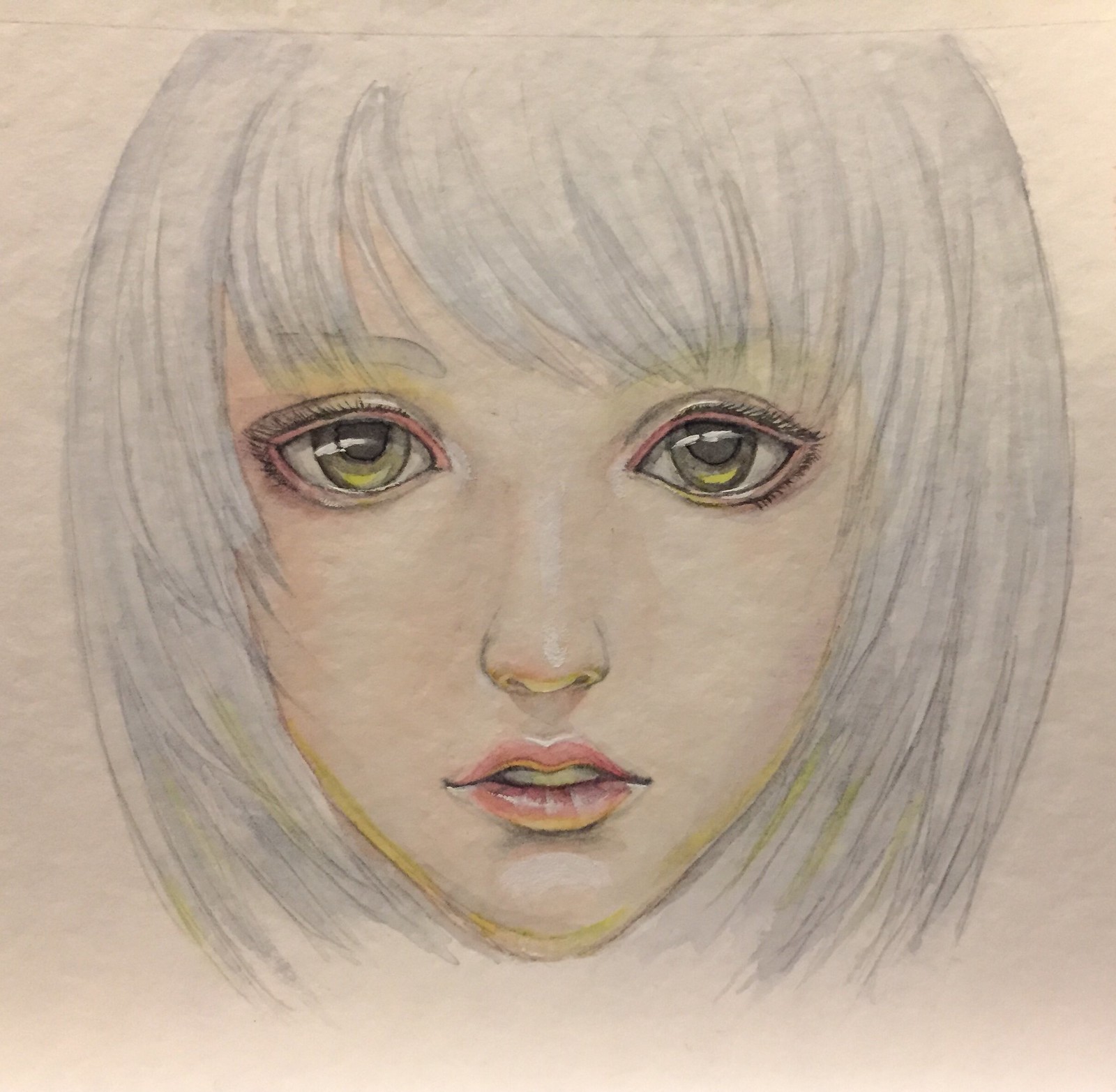This is a highly detailed, sketched and colored picture of a young woman in her late teens to early twenties, created using a combination of colored pencils and possibly pastels or watercolors. The artwork is drawn on a light, textured sheet of paper that appears to be a dusty pink color. The subject has a distinctive heart-shaped face with very fair, pale skin. Her chin-length, blue-tinted hair features bangs that cover her eyebrows, through which they are slightly visible.

She has large, round, mesmerizing green eyes with dark pupils, beautifully outlined with pink eyeliner and mascara. Subtle pink shading is present above her eyes and beneath her chin, adding depth to her delicate features. Her nose is small and delicate, complemented by a bow-shaped mouth adorned with red lipstick, though another observer noted it as pink. Her lips are partly open, revealing a hint of teeth, adding a touch of vulnerability to her expression.

The background comprises minimal but effective blue and black shading, which enhances the contrast and focus on her face. This exquisite, delicately rendered portrait captures the ethereal beauty and detail of the young woman's features, showcasing the artist's skill in blending colors and textures.